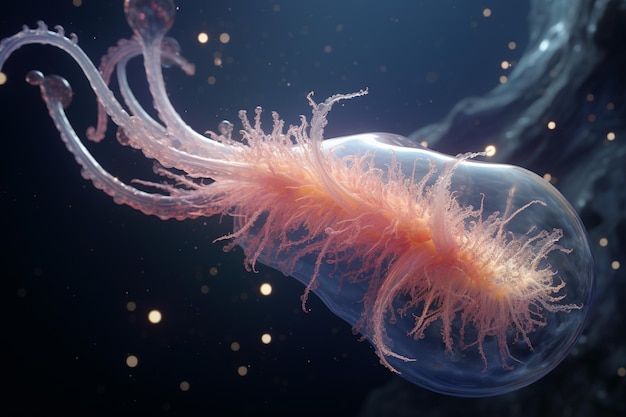A detailed underwater photograph captures a mesmerizing creature, possibly a jellyfish, suspended in a translucent bubble-like structure. This sea animal features numerous long, soft, and hairy tentacles in shades of orange and purple, extending in various directions within the bubble. Additionally, several light blue, almost translucent tails reach towards the upper left, adorned with delicate bumps and ridges. The backdrop of the image is predominantly black, accentuated by scattered yellow and smaller grey dots. Above the creature, a dark blue gradient introduces a touch of brightness to the composition. On the right side, a mysterious green swish ascends towards the top right corner, suggesting a path left by another object or flow in the water. The entire scene is enveloped in an intriguing mix of darkness and subtle reflections, highlighting the ethereal beauty of this underwater marvel.